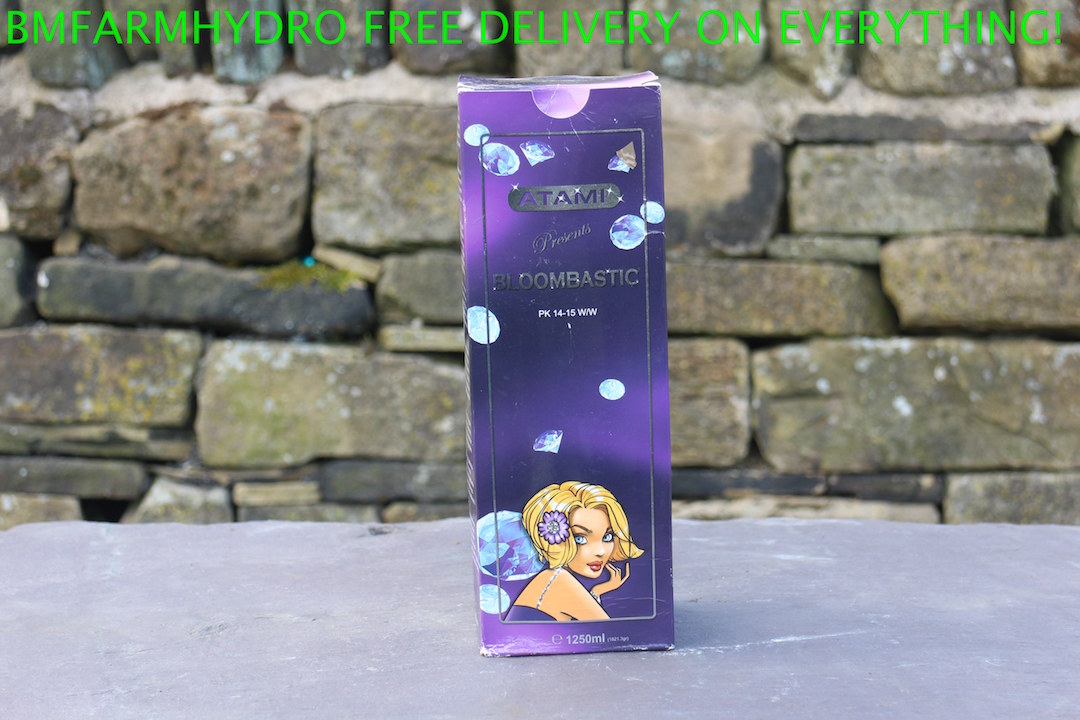The image shows a photo of a package positioned on a gray stone surface. The background features a board made of brown bricks with text that reads, "BMF Farm Hydro - Free Delivery on Everything." The package is a tall, purple rectangular box. At the top of the box, the brand name "ATAMI" is printed, followed by the words "presents Bloom Bastic." Below the text, there's a detailed, animated drawing of a blonde woman with short hair. She has blue eyes and red lips, with a purple flower in her hair. The character is looking forward. The box also features floating diamond illustrations. The package is strikingly vibrant against the neutral-toned background.